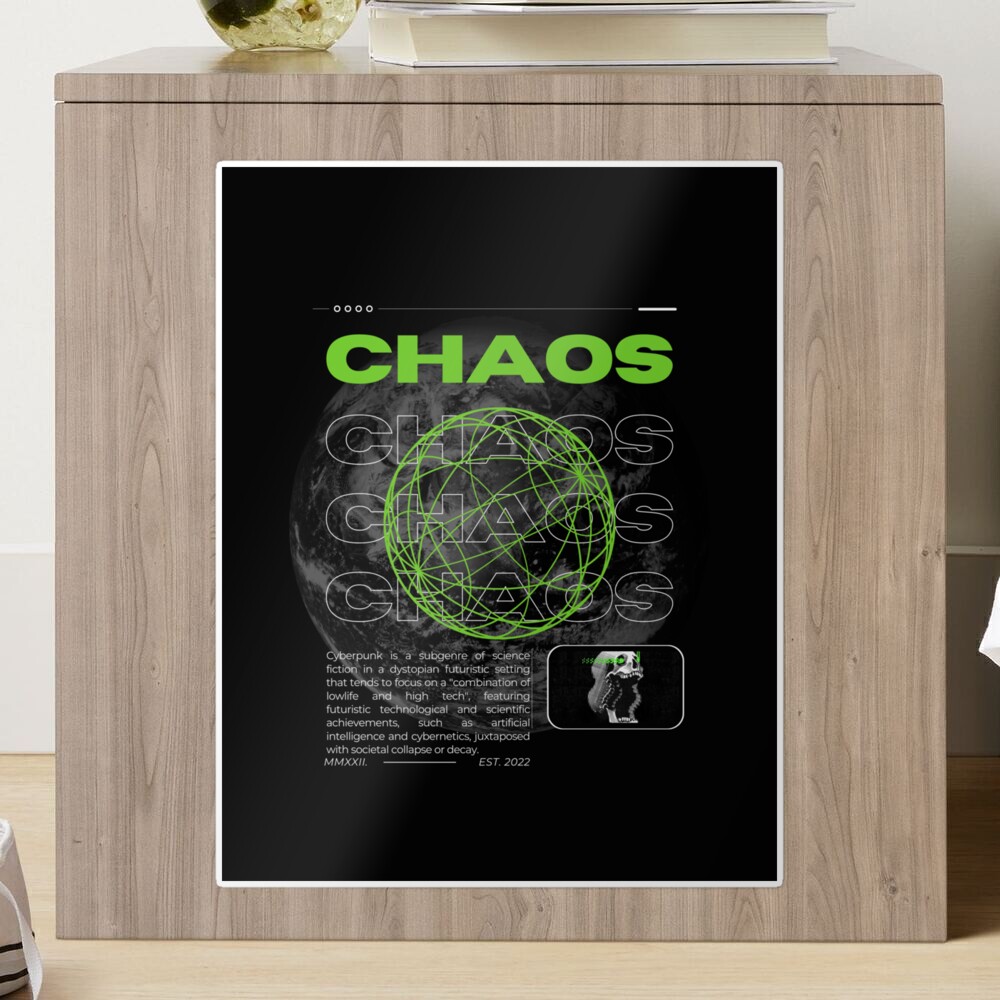This image features a forward-facing view of a wooden box, adorned with multiple objects and sitting on a wooden floor against a blue wall. Sitting atop the light brown wooden box is a slightly dingy glass vase, of which only the bottom half is visible. Adjacent to the vase, positioned to the right, is a book with white pages facing the camera. On the front of the box is a prominent black poster with a white border. Central to the poster is a black background featuring four iterations of the word "chaos"—the first written in dark green, followed by three outlined in white. The poster also includes a green-lined spherical shape resembling a globe and intricate text detailing the definition of cyberpunk, emphasizing themes of high-tech and societal decay, concluded with "MMXII. Established 2022." Additionally, an ominous skull with glowing green eyes and an agape mouth appears on the bottom right of the poster, further enhancing its dystopian theme.